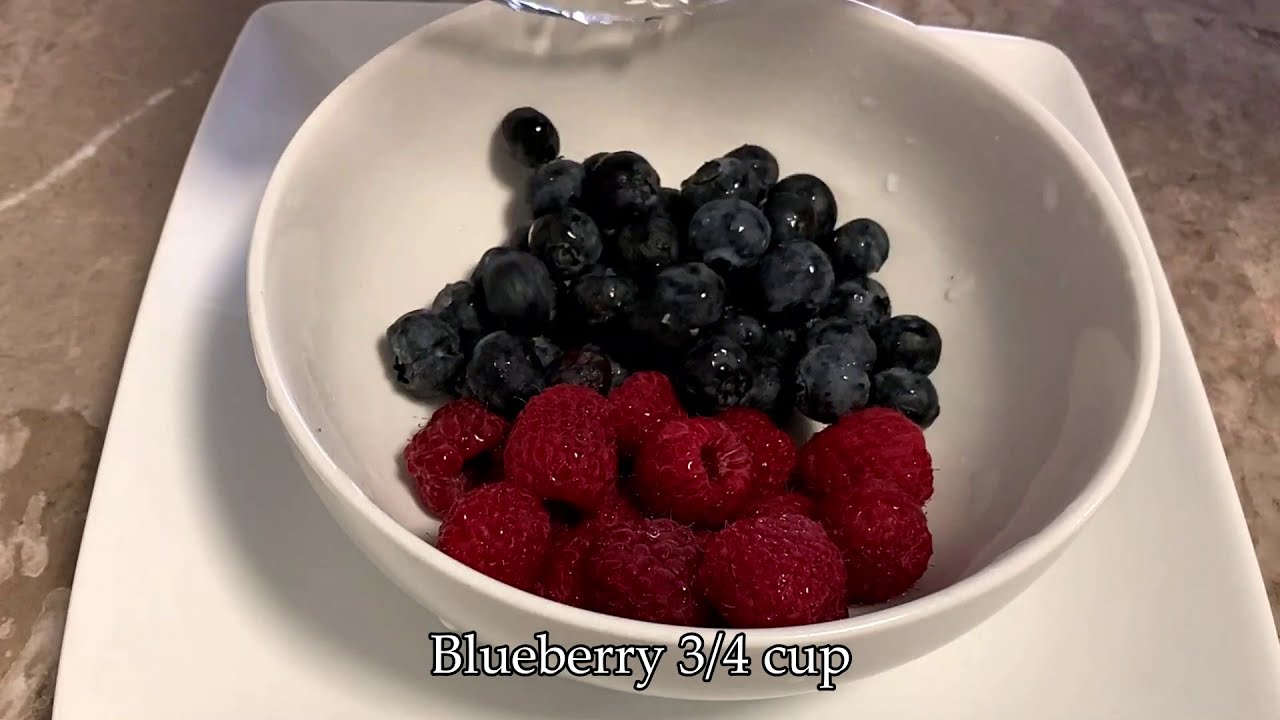In this well-lit kitchen image, a pristine white ceramic bowl sits on a matching square plate atop a pale granite or marble countertop. The bowl contains an abundance of ripe berries, predominantly blueberries on the top half with a generous portion of raspberries on the bottom half, clearly separated within the bowl. The berries are freshly washed, evident from the water droplets clinging to both the fruit and the inside of the bowl. Below the fruit, white text with a black outline reads "Blueberry 3-4 Cup." The shadowing indicates a light source from the lower right, casting subtle shadows on the upper left of the bowl and plate.